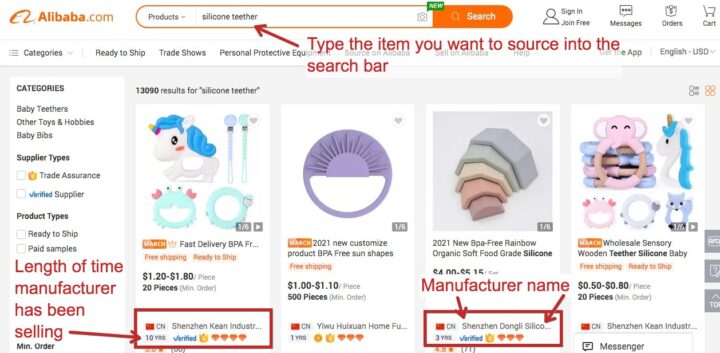The image displays the Alibaba.com website, similar in function to Amazon, serving as a general platform for a wide range of products. In the top-left corner of the screen, the distinct Alibaba logo is prominently displayed. Centered at the top is a search bar where someone has entered a specific product inquiry, highlighted with a red arrow to emphasize its importance in guiding new users on how to initiate a search on Alibaba.

Along the left-hand side, a variety of product categories are visible, allowing users to browse different sections and narrow down their search results. The central area of the screen showcases the search results, displaying various products that match the query.

Each product listing includes detailed information, and boxes highlight key details, such as the length of time a manufacturer has been active on the platform—ranging from over 10 years to as few as one year. The manufacturer’s name is also prominently featured, providing credibility and additional information for potential buyers.

The product images are shown in a gallery format, allowing users to zoom in and view multiple images—such as one item showing six different views. This comprehensive visual and textual layout serves to familiarize first-time users with the functionality and detailed structure of Alibaba.com.